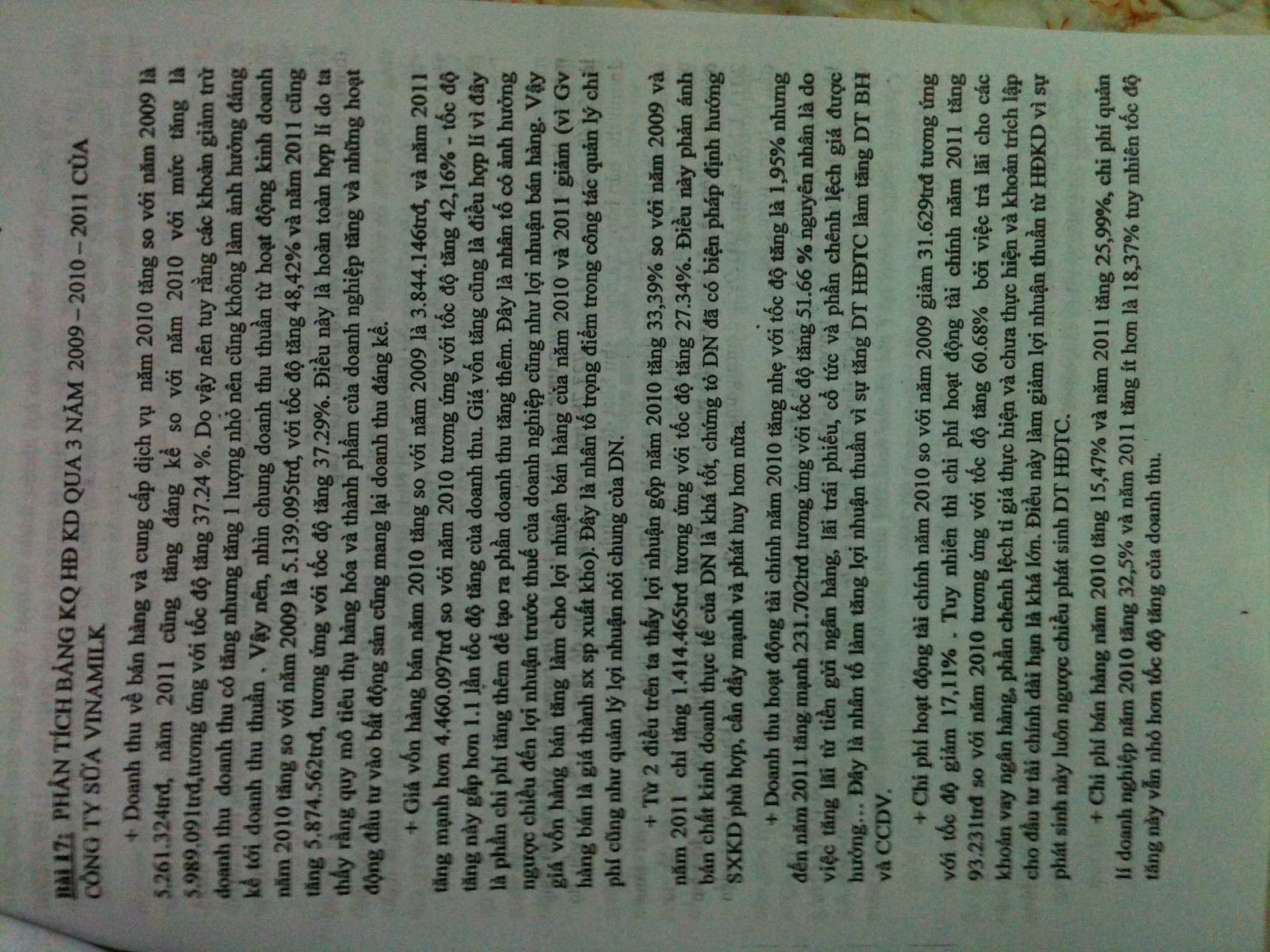This is a horizontal page from a book, visible as if someone turned the book on its side. Although the language, possibly Vietnamese, is not readable, some notable features stand out. The page contains six paragraphs, each starting with a plus sign. The paragraphs are varied in size, with the first being the largest and the second slightly smaller, the rest are roughly equal. The content includes numerous percentages and years, such as 2009, 2010, and 2011, suggesting it might be a scientific article or statistical analysis. The page appears slightly blurry at the bottom, where an indistinct number is present. At the top, there's an unreadable title and an underlined "17". The paper is thin, allowing text from the reverse side to show through, and it might be part of a stapled pamphlet based on its turned-over appearance in the upper left corner.